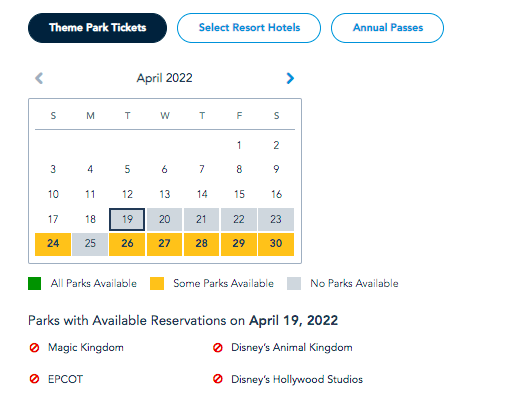This is a screenshot from a calendar application, possibly used for travel planning on an unspecified device. The interface displays three tabs at the top left corner, with the first tab, "Theme Park Tickets," selected. This tab is highlighted with a very dark blue background and white text. To the right are two more tabs: "Select Resort Hotels," featuring blue text with a blue outline on a white background, and "Annual Passes," also with a blue outline and blue text on a white background.

Below the tabs is a calendar for April 2022. The dates from the 19th to the 30th are highlighted. Specifically, the 19th to the 23rd and the 25th are marked with a grey background indicating no park availability for reservations. In contrast, the 24th and the 26th to the 30th have a yellow background, signifying that some parks are available for reservations. There is also a green option for indicating full park availability, but no date within this range is marked green.

The text "Parks with available reservations on April 19th, 2022" appears below the calendar. Each park is listed with a corresponding red circle containing a red line through it, indicating no availability. The parks listed include Magic Kingdom, Epcot, Disney's Animal Kingdom, and Disney's Hollywood Studios.